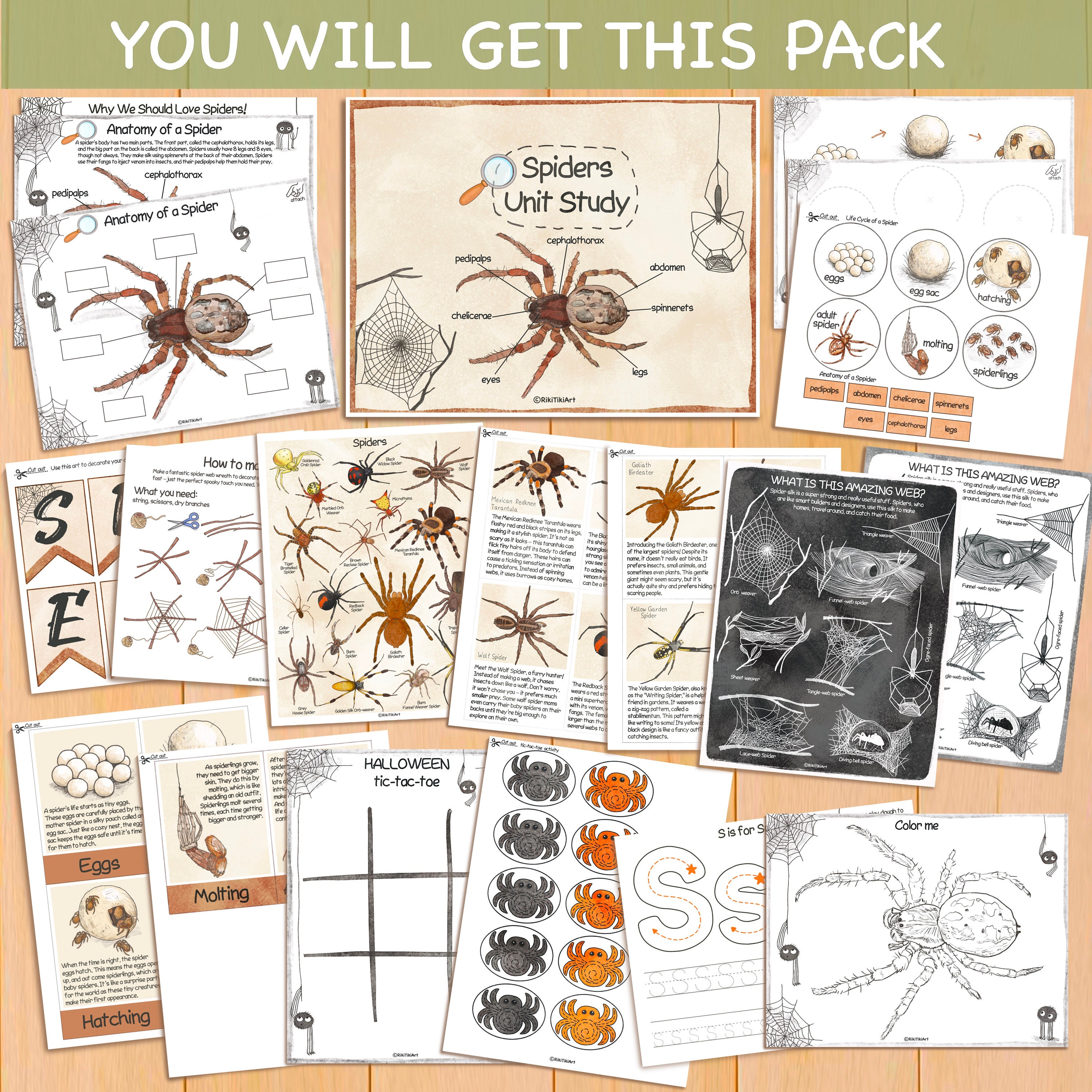This image displays a detailed collage of educational materials tailored for a "Spiders Unit Study", targeting teachers for classroom use. At the top of the collage, a green rectangle with comic sans white text reads, "You will get this pack," emphasizing the bundle's contents. The materials include numerous white, rectangular pages with color graphics, all set against a light brown wood background. The prominently featured contents include detailed illustrations and diagrams of spider anatomy, with labeled parts of various spider species including the black widow, wolf spider, and tarantulas. Accompanying these are practical activity sheets such as Halloween-themed tic-tac-toe, coloring pages, tracing exercises, and stickers. The pack also covers informative topics on different stages of spider life including eggs, hatching, and molting, making it a comprehensive educational toolkit for teaching about spiders.